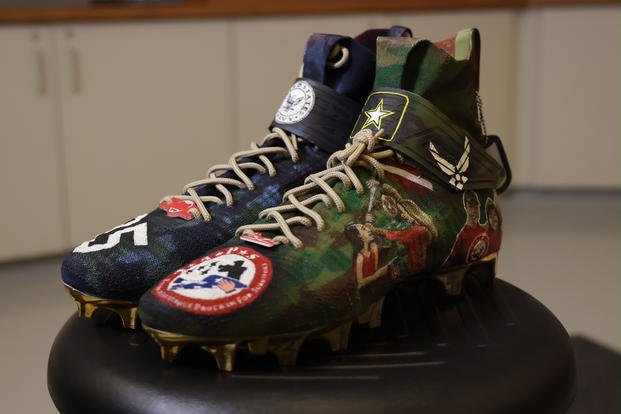The image shows a pair of colorful, camouflage-patterned sports cleats, likely designed for soccer or football, resting on a black leather-topped stool. The cleats feature different military-themed designs: the left shoe boasts a green camo pattern with a U.S. Army logo, while the right shoe has a blue camo design with a Navy logo. Both cleats are equipped with spikes, indicating they are intended for use on grassy fields. Additional details on the green cleat include animated pictures of human figures. The background appears to be a kitchen with several cream-colored cabinets and brown wooden elements.